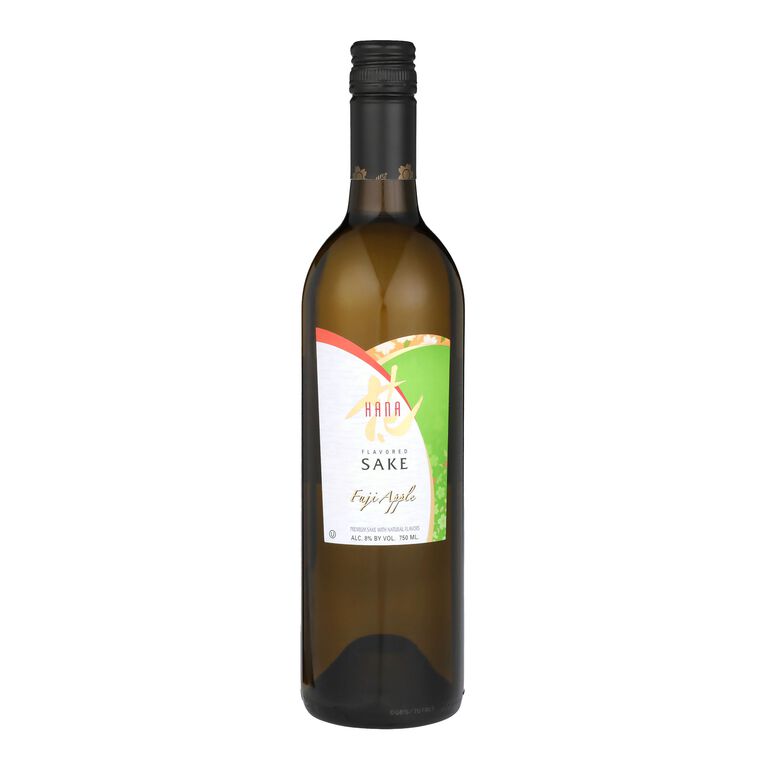This image shows an upright, deep reddish-brown, glossy bottle of flavored sake that resembles a wine bottle. The label prominently features the word "Hanna" in bold letters with "Sake" and "Fuji Apple" written below in script. The background of the label includes subtle apple blossoms and Japanese lettering in yellow gold, creating a visually appealing design with a mix of green, white, red, and gold colors. The bottle is tall and narrow with a screw cap. This Fuji Apple flavored sake contains 8% alcohol by volume, which is higher than most beers. The sake itself is a fermented rice beverage with a unique, appealing appearance, set against a plain white background.